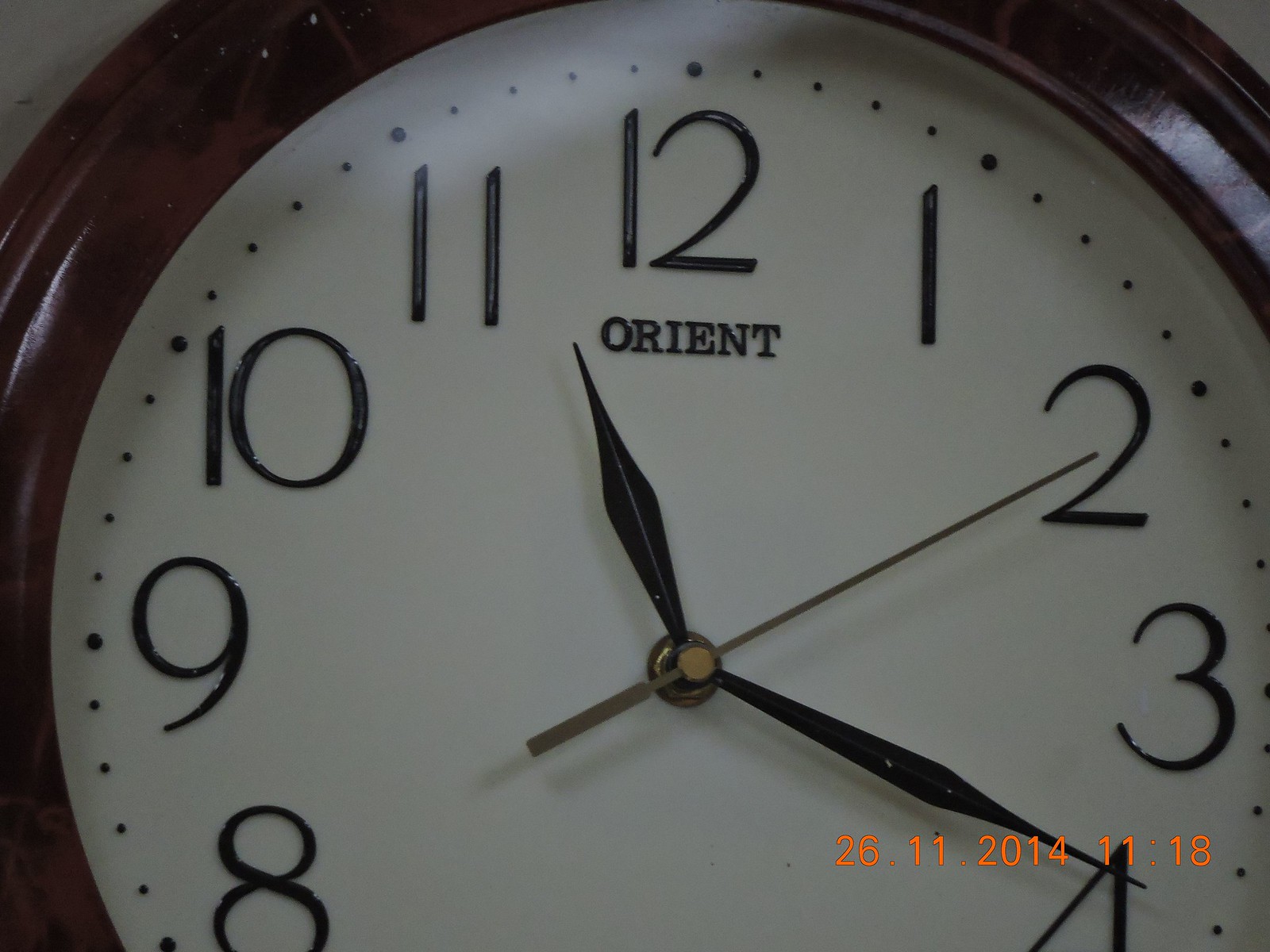A close-up image of a round, wall-mounted clock, featuring a white face and encircled by a dark brown wooden frame. The close-up nature of the photograph cuts off the edges of the clock, partially obscuring some elements. Visible in the image are the numbers 8 and 4, with the latter less prominent as it appears at the bottom edge of the image. The left side of the clock's frame is slightly cropped out. Black numbers clearly mark the hours, and beneath the number 12, the brand name "ORIENT" is positioned. The clock is equipped with an hour hand, a minute hand, and a slender second hand. Additionally, digital numbers displayed at the lower right corner of the clock read "2-26," "11-2014," and "11-18," which could represent dates or times, adding to the clock's functionality and aesthetic.